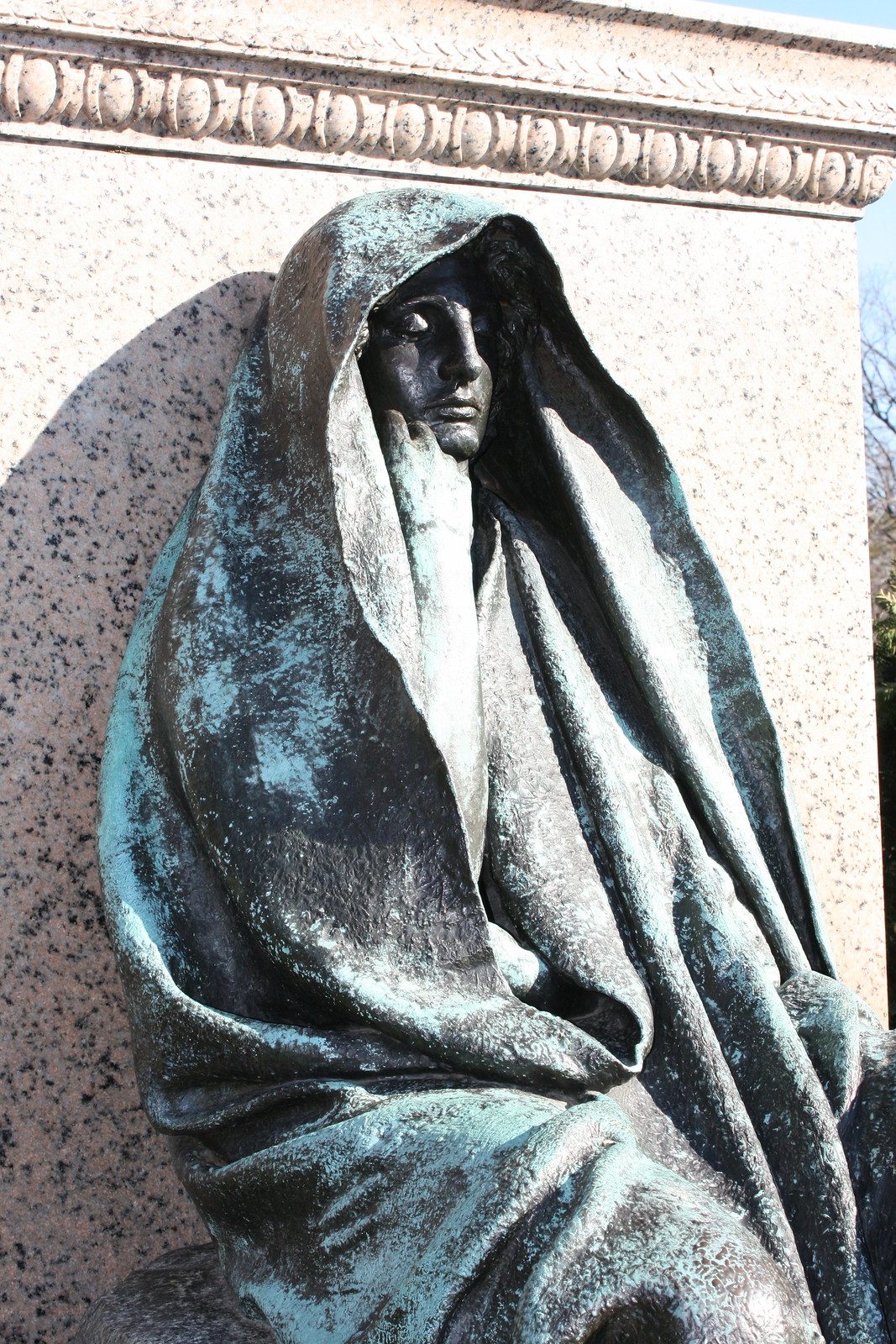The image features a detailed, weathered statue of a figure cloaked in a blanket, seated against a stone wall with intricate borders at the top. The statue, likely made of bronze or copper, displays a blackish-brown hue with weathered green spots scattered across its surface. The figure, whose gender is ambiguous, sits with their right arm supporting their chin, their closed eyes and nose visible beneath the hooded cloak that envelops their entire body. The serene posture suggests a meditative or prayerful state. The background reveals a spackled stone wall with variations of light and dark brown, set against a clear blue sky with barren trees and sparse bushy vegetation to the right, further highlighting the tranquil, contemplative atmosphere of the scene.